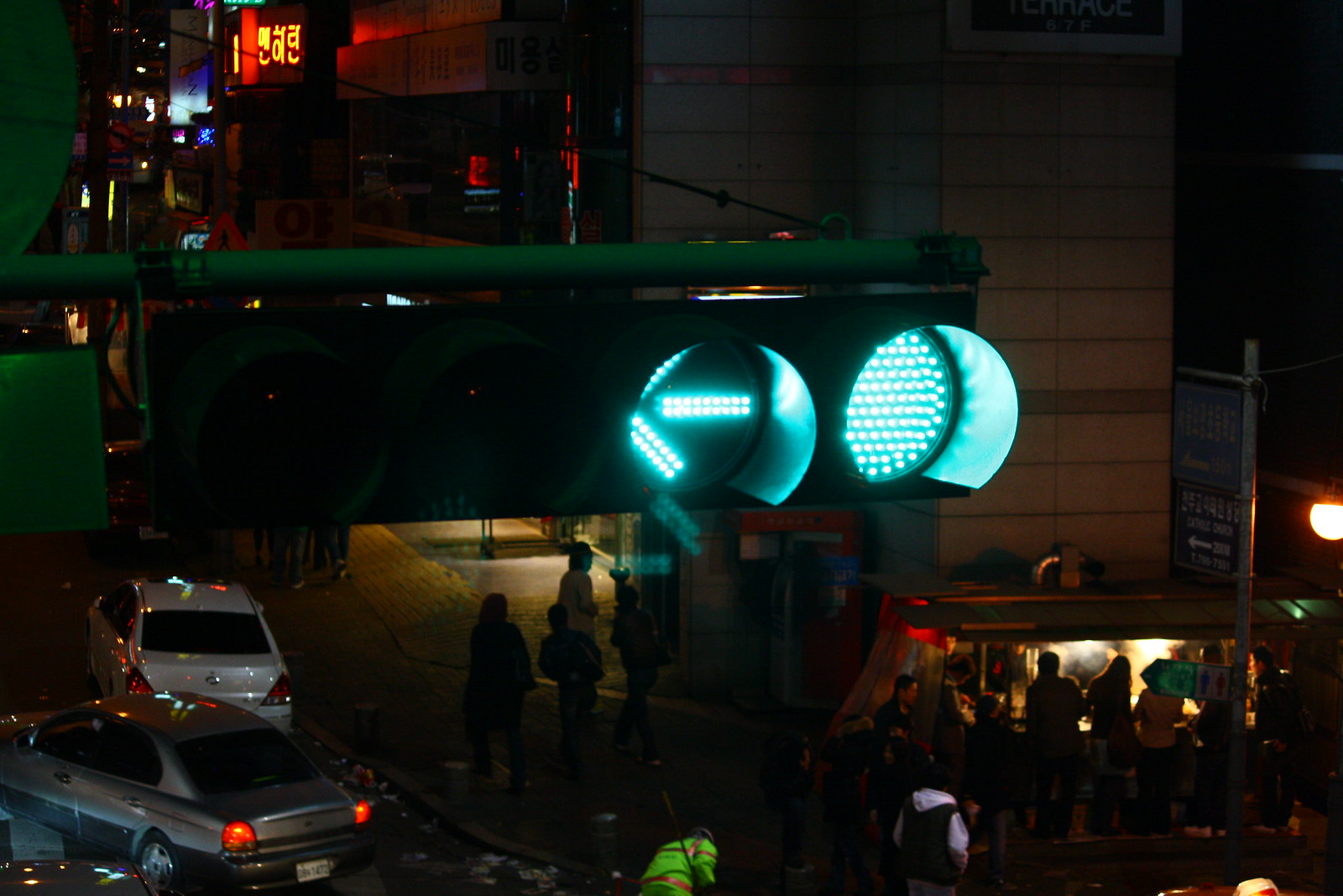This image captures a bustling nighttime city street corner. Dominating the foreground is a traffic light with a close-up view showing its top green light illuminated, as well as a left turn arrow light. The traffic light stands out prominently with its four rows of lights, all affixed to a green pole. Below the traffic light, in the bottom left corner, there is a vibrant food stall or merchant stand with bright lights and people gathered in front of it. Behind the stall, a tall building rises up, with windows visible starting from the third floor. 

In the left part of the image, the street curves around the corner, and silhouettes of four pedestrians are visible against the city lights. The bottom left also features a couple of cars, including a parked white car and another navigating around it. Extending from the left to the center of the image and into the background, a series of buildings adorned with neon signs add to the urban night scene. The whole image is filled with the energy of city life, with about 20 people dispersed throughout the frame, though their features are obscured by the backlighting. The street is lively, with a mixture of people walking and cars maneuvering through the neon-lit roads.